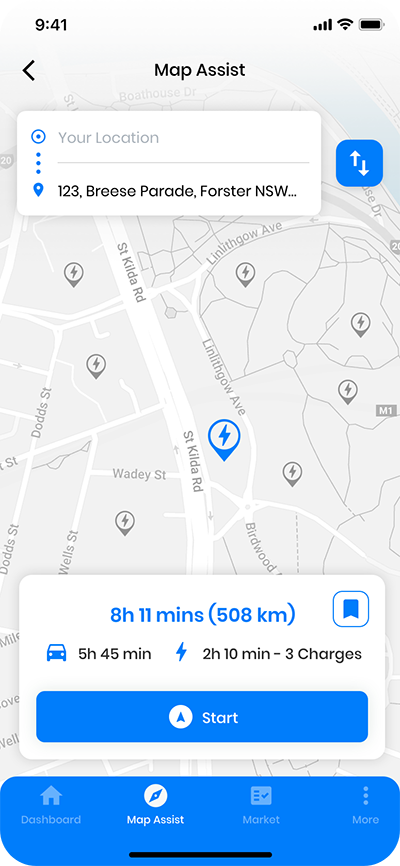A screenshot of a map application taken at 9:41 displays a fully charged battery icon. The top-left corner reveals the time and battery status. Below, the screen reads "Map Assist" in black text. A white pop-up box at the top indicates "Your location," followed by a gray horizontal line. The location is listed as "123, Breese Parade, Forster, NSW." To the right of this address, a blue square with rounded edges features white arrows pointing up and down.

The background shows a grayscale map with a vertical road running north to south and several intersecting streets. Several locations are marked, including a prominent blue circle with a lightning bolt icon and a downward-pointing triangle, along with similar gray icons.

At the bottom, a white rectangle contains blue text saying "8 hours 11 minutes" and "508 kilometers," detailing a drive time of 5 hours and 45 minutes, 2 hours and 10 minutes for three charging stops. A blue "Start" button and a white circle with a direction icon are also visible at the bottom.